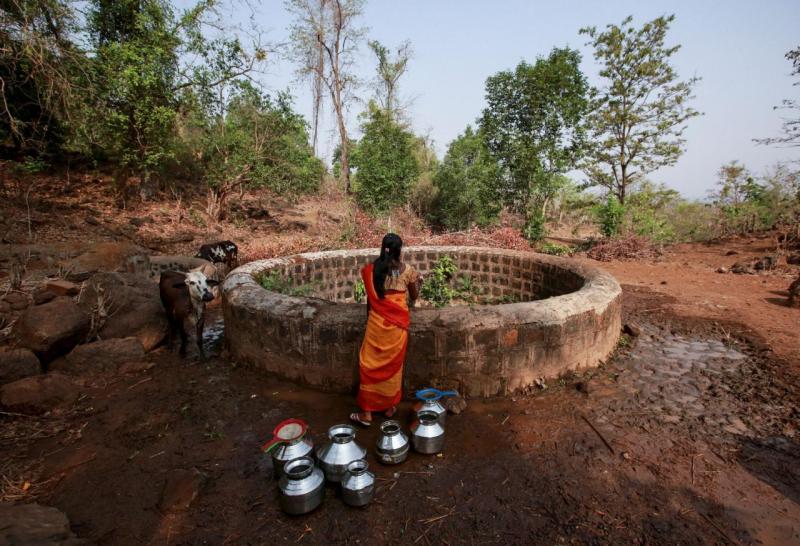This rectangular photograph captures a vibrant outdoor scene under a bright blue, sunny sky. Centering the image is a large, circular structure resembling a well, crafted from an assembly of large mudstones and mortared stones, with plants emerging from within it. A young woman, possibly from South Asia, stands with her back to the camera at the edge of this well. She is dressed in an orange and red sari, with her waist-length black hair pulled back. Behind her, seven metal jugs and strainers suggest she is collecting water. The scene also features two cows; one brown and white cow stands next to the well, while another is visible in the background. The ground near the well is saturated and muddy, transitioning to a drier, reddish-brown soil farther away. The backdrop is lush with trees and varied vegetation, adding to the natural beauty and authenticity of this rural setting.